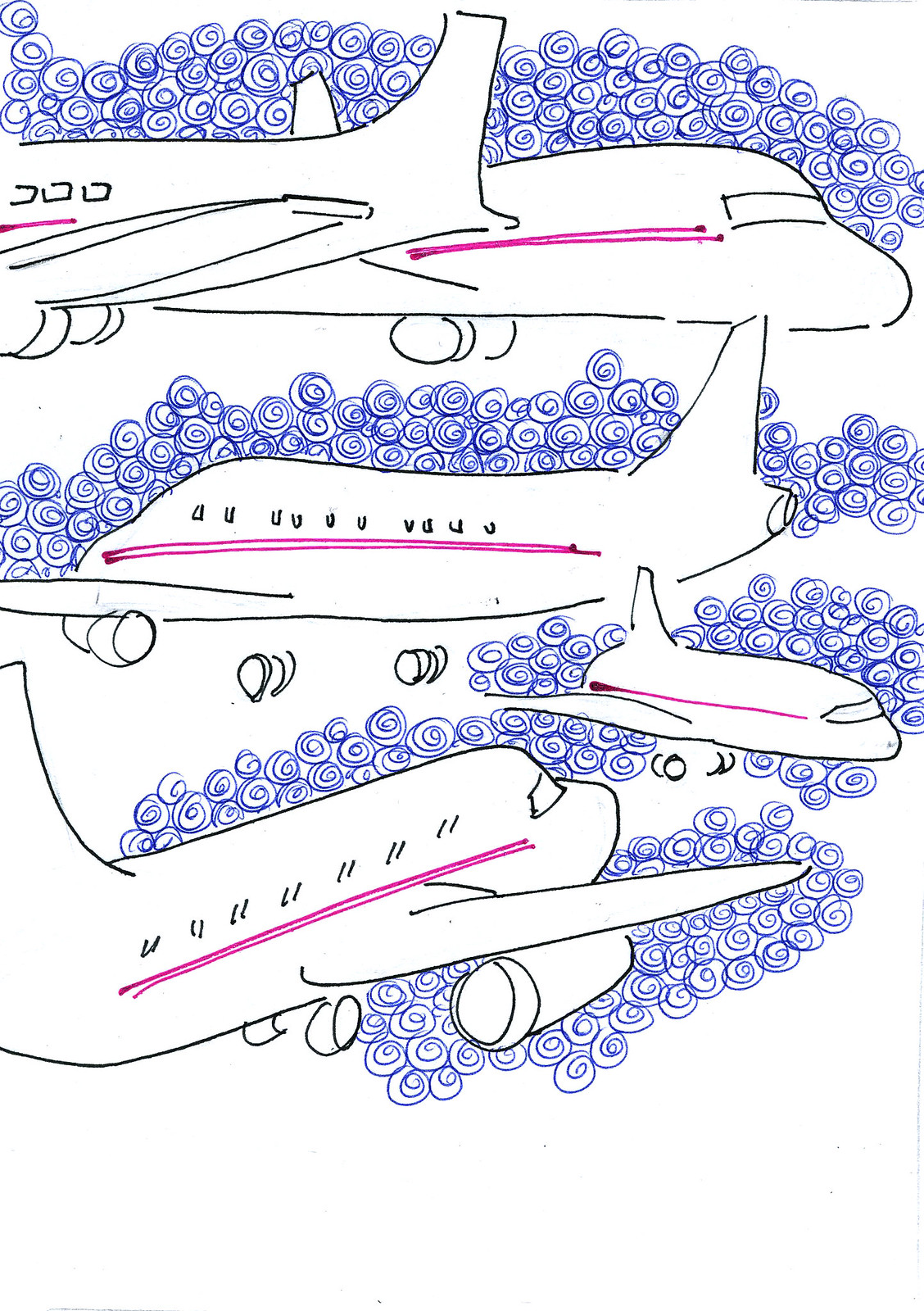This image showcases a hand-drawn assortment of five stylized airplanes, possibly representing different viewing angles of the same aircraft or different planes altogether. Each airplane is outlined in black and decorated with a series of red or pink stripes extending from the cockpit to the tail over a predominantly white body. Small windows run along their sides, accompanied by a large front-facing window on the airplane's nose. Each plane features landing gear, indicative of them being mid-flight.

The airplanes are depicted within a dynamic blue ink backdrop, with swirling lines representing the sky surrounding each aircraft. The composition details the positioning of these planes: the topmost airplane's nose points to the right, partially cut off just past the wing; another airplane in the midsection faces left, appearing slightly as if it's flying away with its tail end visible; below it, a smaller plane angles to the right; another aircraft in the bottom left flies rightward, seemingly towards the smaller plane. Finally, there's a plane at the very bottom with its cockpit directed upwards and right, presenting a view of its right wing extending outward.

Overall, the drawing displays a whimsical assembly of airplanes in different orientations, cohesively bound by the blue, sky-representing swirls that trail behind and encapsulate each plane.